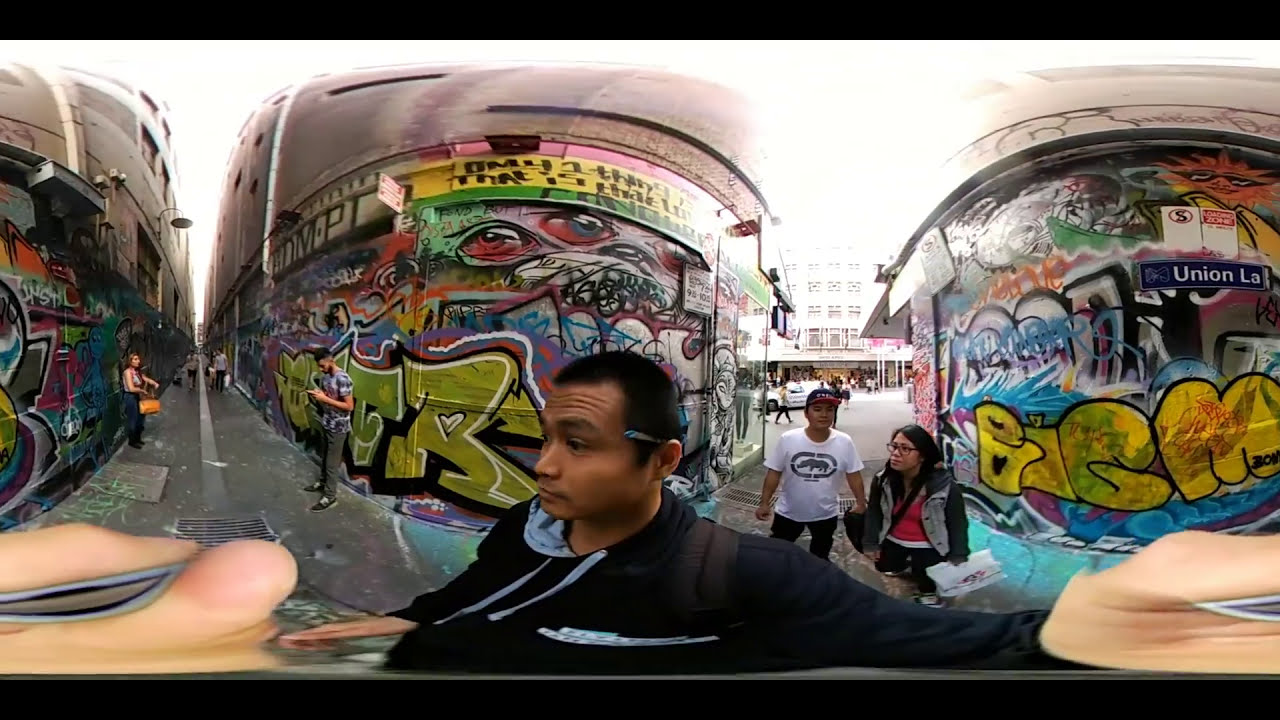In this dynamic wide-angle photograph, a young man with an olive complexion, short black hair, and a black hoodie featuring gray inner lining and drawstrings stands prominently in an alleyway seemingly filled with vibrant energy. The man is notably carrying a pencil behind his ear and appears to be gesturing with his hands while looking to his right. His dark hoodie contrasts with the brightly colored, graffiti-covered walls of the alleyway surrounding him. The street art, adorned with large, stylish letters and images, blankets the three large structures behind him, each topped with silvery domes that resemble old, massive ships or buses parked amidst the urban sprawl. One structure bears the letters "B-I-B-M" while another displays a large "F" and "R." To the far right, a blue street sign reading "Union Law" is visible. The bustling market area is populated with various people; to his right, a lady dressed casually and a young man in a white t-shirt can be seen, while figures of pedestrians, shoppers with bags, and cars in the background add to the lively ambiance. The alleyway itself seems like a portal opening into the crowded, colorful streets beyond, capturing the essence of an energetic marketplace.